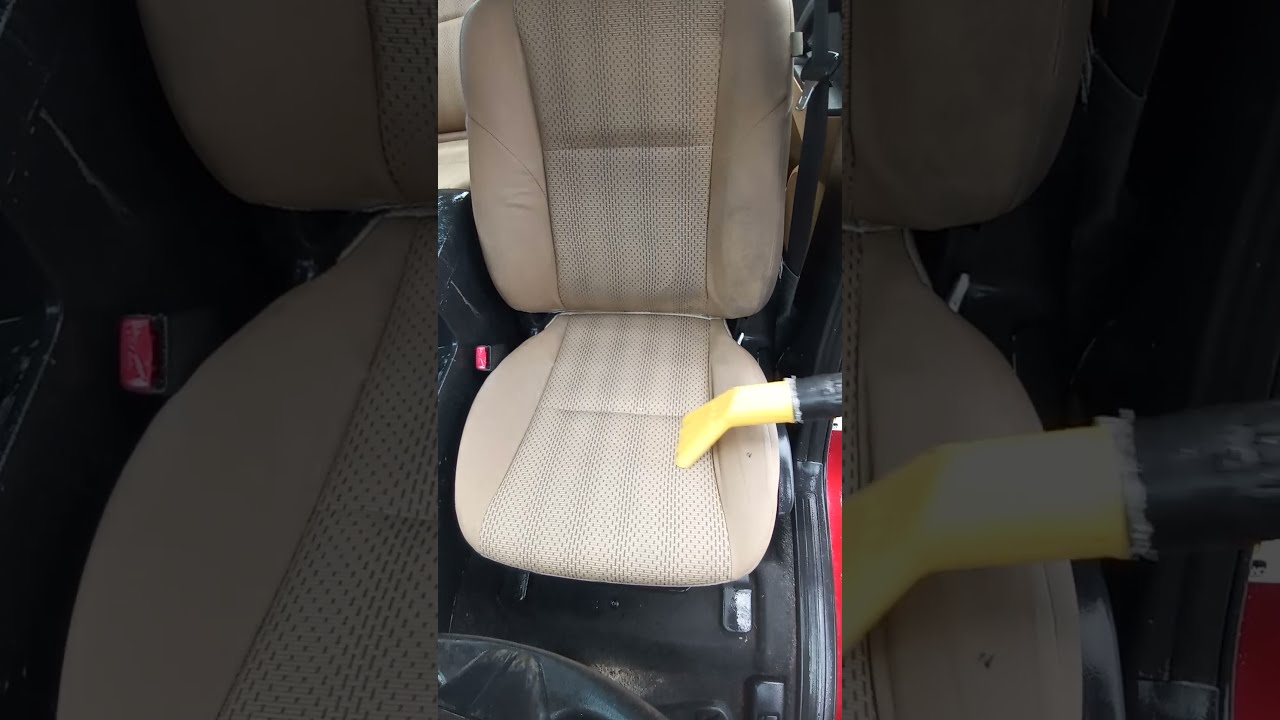This image is a detailed view of a car interior, focusing on a cream-colored car seat being vacuumed. The primary photograph in the center is a vertically oriented snapshot capturing a slightly dirty beige cloth car seat with visible black marks from years of use. A yellow-tipped vacuum nozzle can be seen intruding from the right side, actively suctioning dirt and debris from the seat. The seat has a black floor beneath it, and a seat belt buckle with a red button is noticeable on the left side if sitting in the seat. The overall image is a horizontal rectangle, with the central photo flanked by darker, zoomed-in sections of the same car seat, emphasizing the cleaning process. There is a hint of carpeting with some dirt at the bottom, suggesting the cleaning might extend to the floor next. The aspect ratio and format suggest this might be a screenshot from a social media reel, possibly TikTok or Instagram, capturing the interior detailing process of what could be a minivan or passenger car.